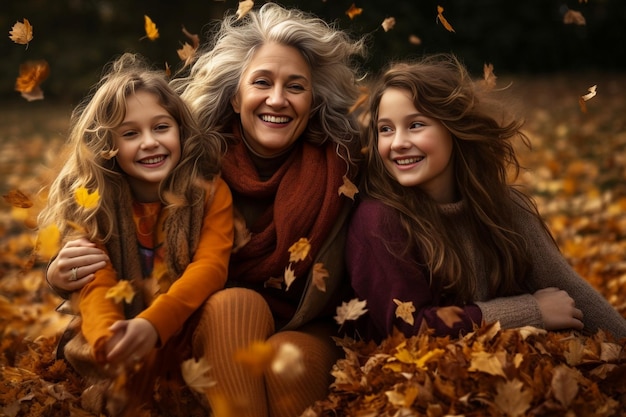This vivid, high-quality photograph captures a joyous autumn moment featuring three females—a middle-aged woman and two young girls—sitting amidst a large pile of orange and brown fallen leaves. The image is taken in landscape mode, focusing on the trio centrally. The middle-aged woman, with gray hair and a large smile, sits in the center wearing tight yellow pants, a jacket, and a maroon scarf. She has her right arm lovingly wrapped around the young girl to her left, who appears to be around 10 years old, while the girl on her right, approximately 13 or 14 years old, looks towards her. Both young girls have long, wavy hair, and the three of them are dressed in fall shades of orange, yellow, and burgundy. The wind is blowing, and leaves are seen both falling in the background and swirling around them, adding to the dynamic, fall ambiance. The scene exudes warmth and familial love, with everyone's face illuminated by genuine smiles.